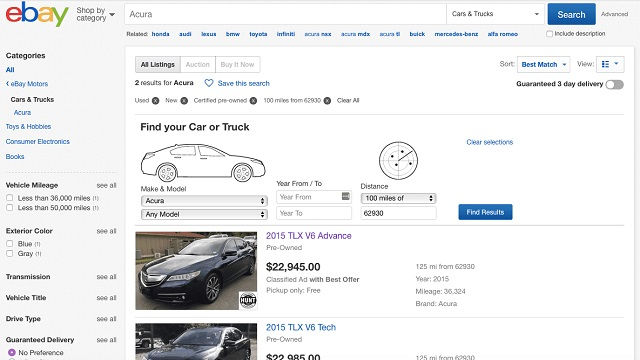The screenshot captures an eBay search result page for a car query. The interface appears on a gray background, prominently featuring the iconic eBay logo in the top left corner, with "e" in red, "b" in blue, "a" in yellow, and "y" in green. Below the logo, the category "Shop by category" is selected, revealing filters for "Acura" under "Cars and Trucks."

The search specifies a distance of 100 miles from the 62930 zip code, though no specific model years have been chosen. Additionally, a highlighted section encourages users to "find your truck."

The first search result displayed is a detailed listing for a black 2015 Acura TLX V6 Advance sedan, shown from a front side angle. The ad specifies that the vehicle is pre-owned, listed at $22,945 as a classified ad with a "best offer" option. The sale is "pickup only" and free, with the vehicle located 125 miles from the provided zip code. Further details reveal the car has been driven 30,324 miles.

Below, a partially visible image shows another black sedan, seen from the side. The description beside it notes a 2015 Acura TLX V6 Tech model, also pre-owned, listed at $22,985. Similar to the first listing, this vehicle is located 125 miles from the search area, though the complete zip code is truncated.